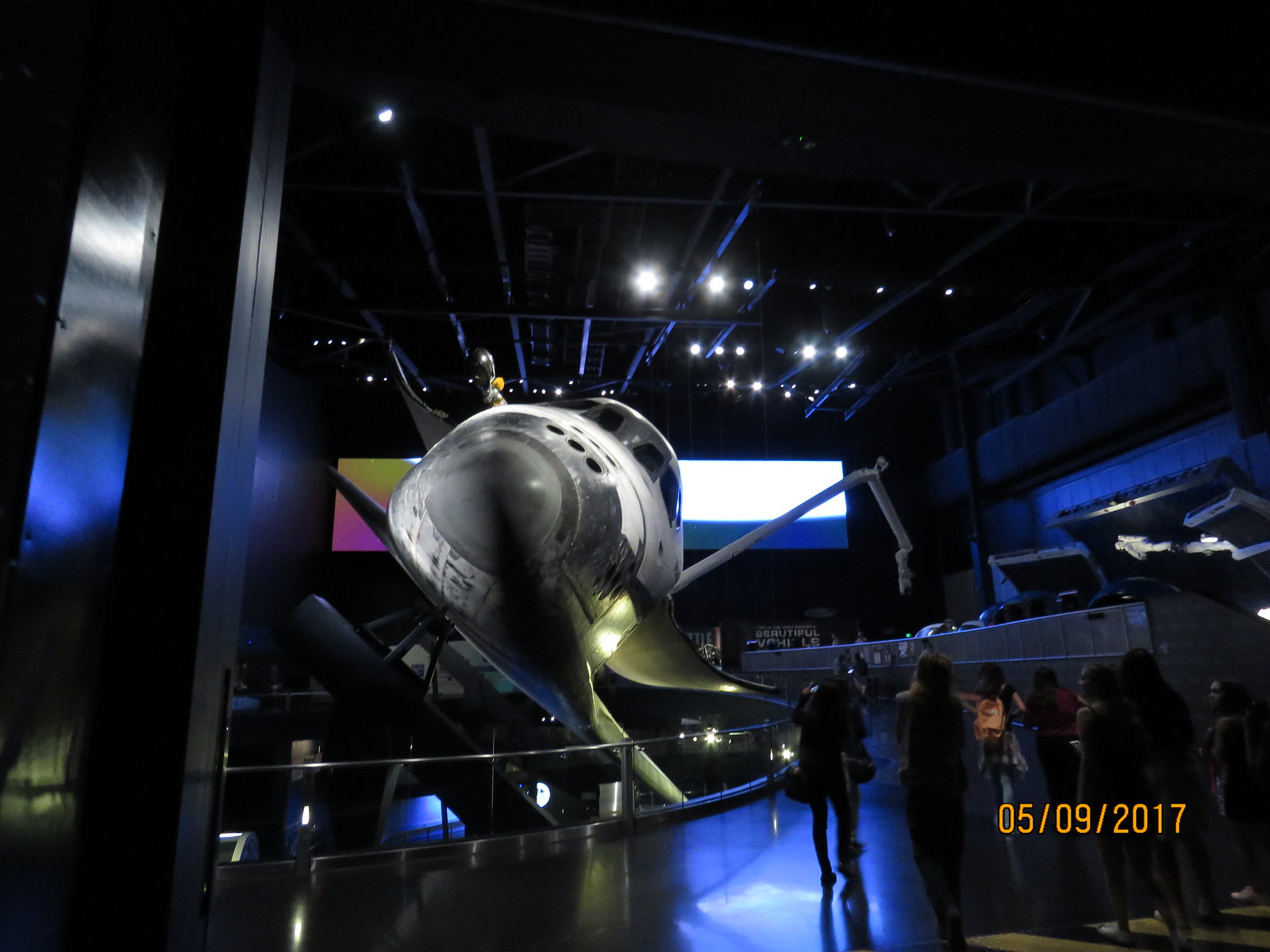This image features a predominantly black background, suggesting it was taken at night. At various points within the composition, vibrant blue and silver elements catch the eye. A series of bright white lights illuminate parts of the scene, enhancing the nighttime ambiance. In the lower right corner, an orange timestamp reads "05-09-2017." The image's content remains ambiguous, but the interplay of colors and lights creates a striking visual effect.